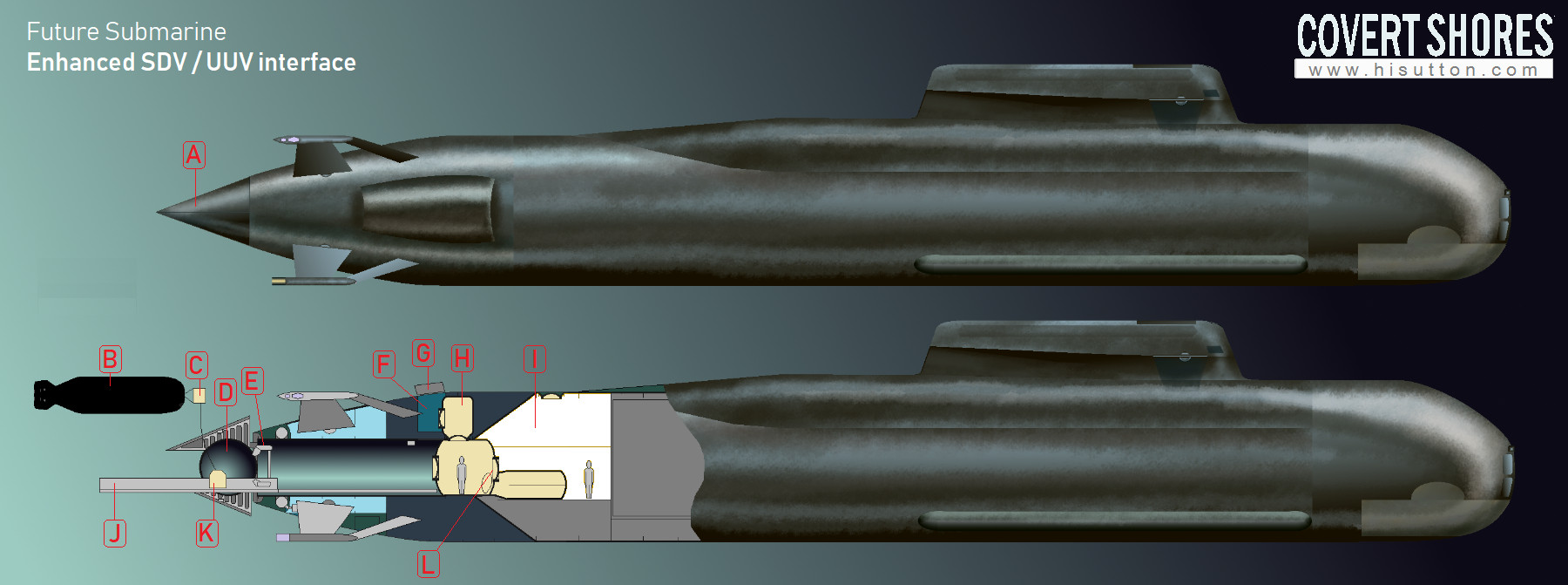The poster titled "Future Submarine Enhanced SDV/UUV Interface" features a detailed, narrow landscape illustration of a futuristic submarine. In the top left corner, the title is written in white, while the top right corner displays "Covert Shores" in uppercase white letters and the website "www.highsutton.com" below it.

The poster showcases two versions of the submarine: 
- The top image presents an exterior view of the entire submarine, which has a conical tail end, resembling a bomb.
- The bottom image provides an internal diagram, focusing on the left part of the submarine. It reveals various internal components, including a round sphere, a tube, and a couple of crew members. The internal elements are labeled with the letters A through L in red, though there is no legend explaining these labels.

The background transitions from blue on the left side to teal green on the right side. The detailed labeling and distinct background colors make the poster both informative and visually engaging.